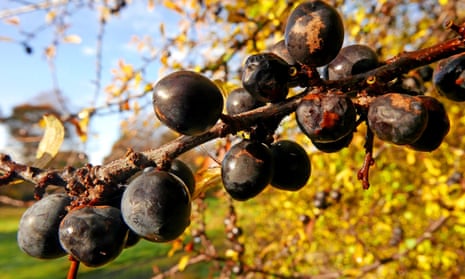This close-up daytime image features a dynamic branch extending from the upper right to the lower left, curving slightly upwards towards the center. Adorned with numerous dark black berries, the branch displays a striking contrast between its healthier, more robust berries clustered towards the bottom, and the decaying ones with reddish, irregular spots towards the top. To the right of the image, a tree stands in the blurry background, with green and yellow leaves intermingling amongst additional bunches of similar black berries. On the left side, the distant blue sky meets a stretch of green grass at the bottom, creating a serene outdoor setting. The backdrop remains out of focus, emphasizing the intricate details and textures of the foreground branch and berries.